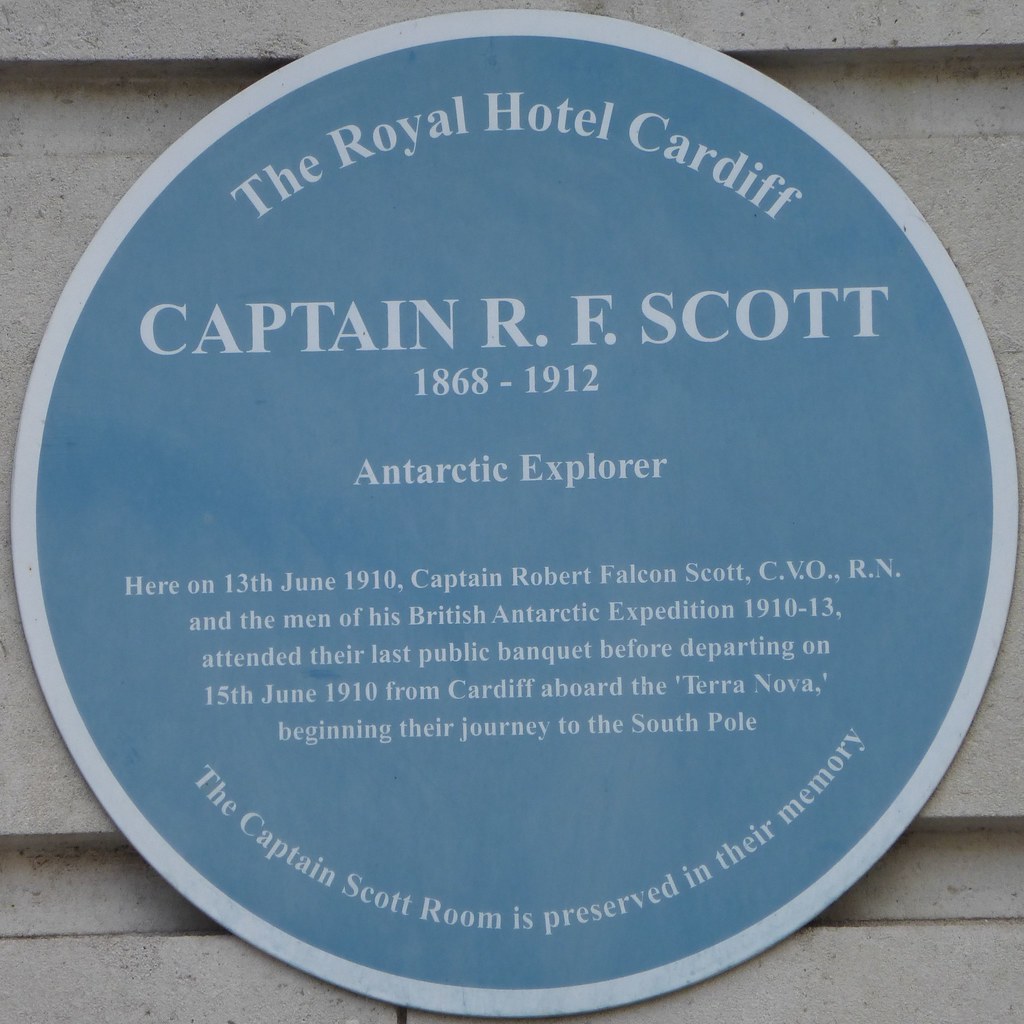In this image, we see a circular sign attached to the side of a building. The sign, which has a white ring around its edge and features white print on a lighter blue background, commemorates an important historical event. It reads: "The Royal Hotel Cardiff. Captain R.F. Scott, 1868-1912, Antarctic Explorer." The plaque details that on June 13, 1910, Captain Robert Falcon Scott, CVO, RN, along with the men of the British Antarctic Expedition 1910-1913, attended their last public banquet at this location before departing on June 15, 1910, from Cardiff aboard the Terra Nova, embarking on their journey to the South Pole. Furthermore, it honors Captain Scott's memory by noting that the Captain Scott room is preserved in their memory. 

This plaque serves as a tribute to Captain Scott's significant contributions and the ultimate sacrifice he and his team made in their quest for Antarctic exploration.